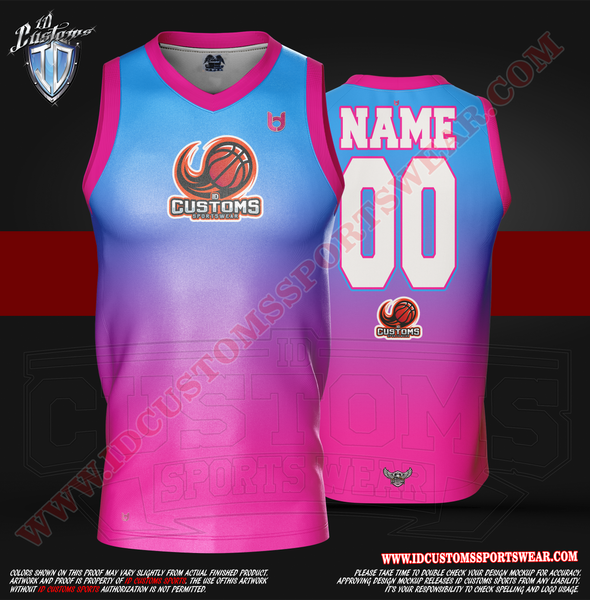This image is a detailed digital mock-up of a customizable sports jersey, prominently featured as an advertisement. The sleeveless jersey showcases an ombre color scheme, transitioning from light blue at the top to vibrant pink at the bottom, with a hint of purple in between. The neckline and armholes are trimmed in bright pink. The front of the jersey displays a dynamic logo of a flaming basketball along with the text "Customs Sportswear." 

On the left chest, there’s an additional logo, and the back of the jersey is designed to feature the player's name and number in white, outlined with pink – in this instance displaying "NAME" and the number "00." The background of the image is a two-tone black with a central red stripe running through it. A watermark of the website "www.idcustomssportswear.com" is visibly spread across the entire image. 

Accompanying the visual design, there is important textual information at the bottom, advising viewers to take the time to double-check their custom design for accuracy, as the approval of the design mock-up releases ID Customs Sports from any liability. It highlights the responsibility to verify spelling and logo usage.